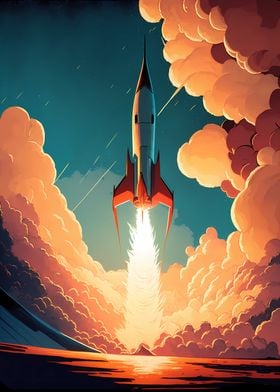This digitally produced artwork depicts a rocket ship launching upwards from the center of the image, with vibrant fiery oranges and reds emanating from the base of the rocket. The rocket's body has a red base, a silver midsection, and a black tip, creating a visually striking contrast against the dark blue dusk sky. Plumes of smoke billow out from both sides of the rocket, showcasing a gradient of dark colors that transition into lighter hues, resembling a sunset. At the very bottom of the image, there appears to be a reflective surface, possibly water, capturing the light and colors from the rocket's fiery exhaust. The smoke surrounding the rocket seems almost bubble-like, with muted orange and reddish tones, adding to the dynamic and atmospheric composition of the scene.